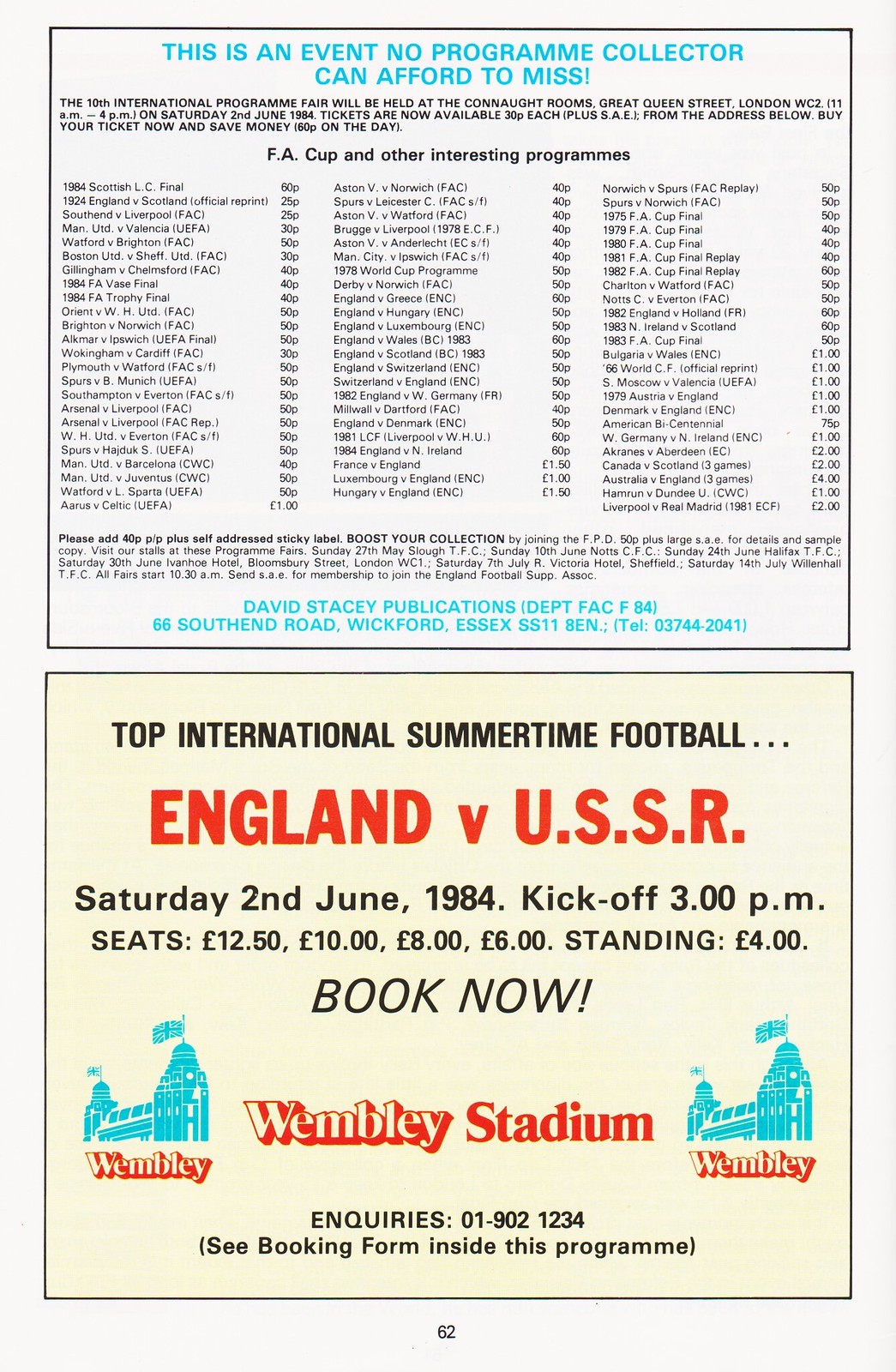This detailed page, page 62 from an official game day program, is divided into two halves and features essential information for soccer enthusiasts and program collectors alike. The top half is an advertisement for the 10th International Program Fair, a must-attend event for collectors, to be held at the Connaught Rooms, Great Queen Street, London, WC2, on Saturday, 2nd June, 1984, from 11 a.m. to 4 p.m. Tickets, available now for 30p each plus an SAE, can be obtained from David Stacey Publications, Department FAC, F84, 66 South End Road, Wickford, Essex, SS11. Alternatively, tickets can be purchased for 60p on the day. The advertisement also highlights the variety of programs available, including the F8 Cup, with prices ranging from 25p to 4 pounds.

The bottom half of the page features another advertisement, this time for a significant soccer match: Top International Summertime Football between England and the USSR, scheduled for Saturday, 2nd June, 1984, with a kickoff at 3 p.m. The ad provides ticket prices for seats (ranging from 12.50 pounds to 6 pounds) and standing (4 pounds), and urges immediate booking at Wembley Stadium. Wembley's iconic image is depicted on both sides of the page with "Wembley" written underneath it, and further inquiries can be made by calling 01-902-1234, with a booking form available inside the program.